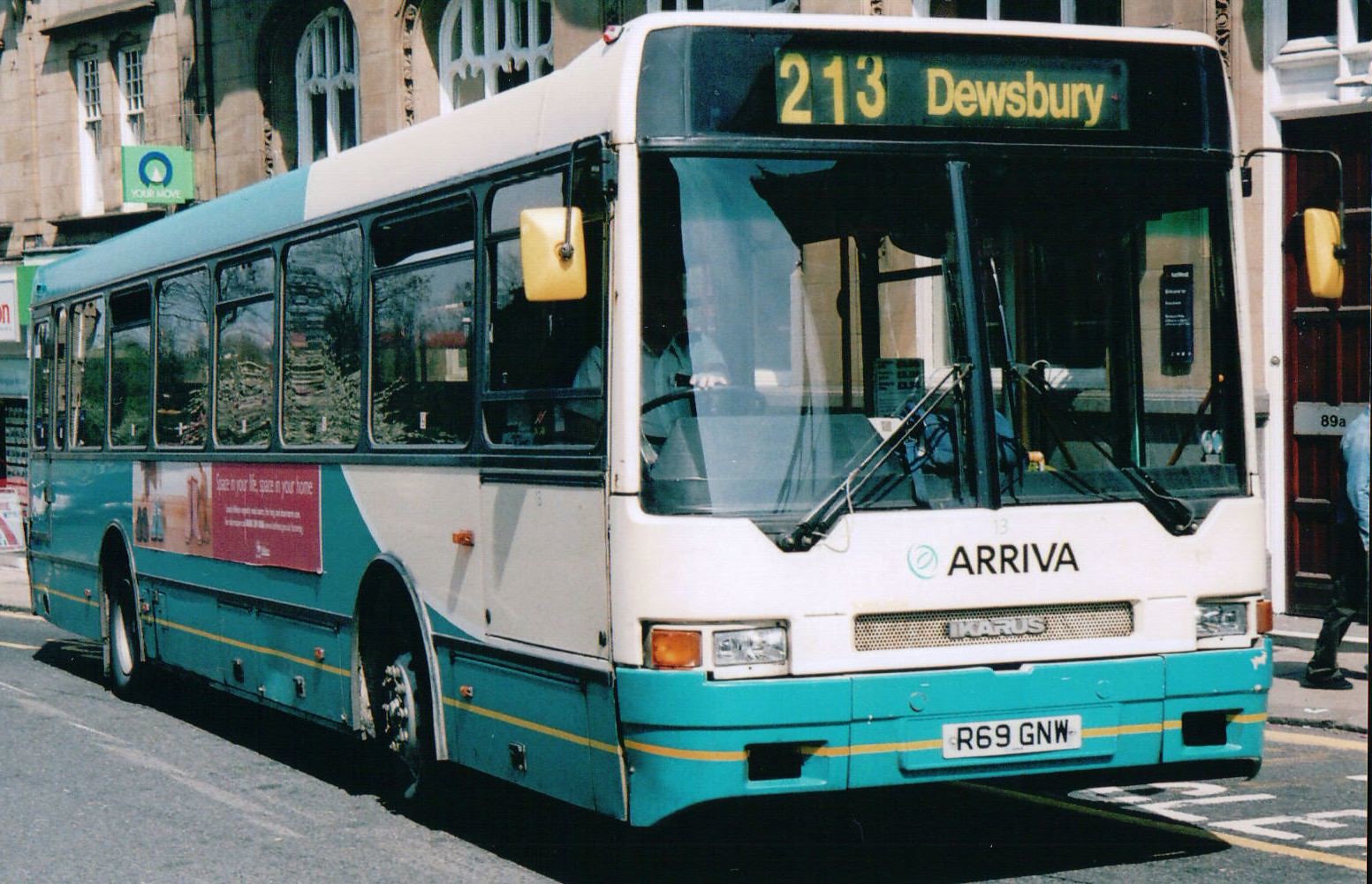The photograph captures a transit bus navigating a city street, prominently featuring a white and teal color scheme. The bus is angled, with the front facing slightly towards the right and the back extending to the left. The front of the bus displays a black window section with a yellow sign above reading "213 Dewsbury." Below the windshield, the name "Arriva" is visible in black font, and further below, a white rectangular license plate bears the number "R69GNW." Notably, the bus's body transitions from white at the front to teal towards the back, and includes dark black windows along its length. An advertisement on the side of the bus includes a red panel with part of the text visible stating, "space in your life, space in your home," though the rest is too small to discern. Strikingly, the image gives the illusion that one of the bus's tires is missing, which could be an optical trick. In the background, a tall, cement building with white-framed windows is partially visible, against a grey street providing the setting for the scene.